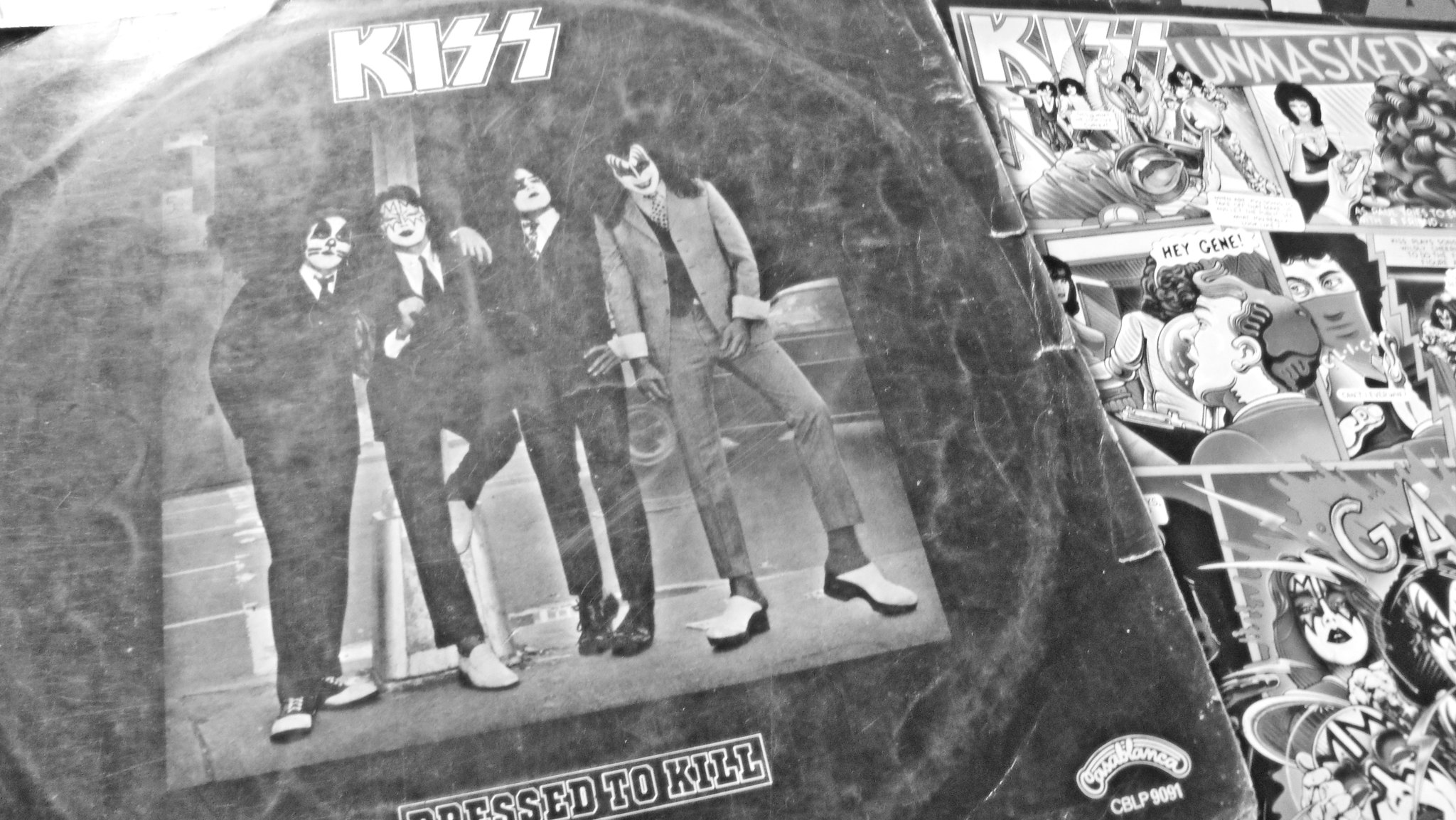This classic black and white photograph serves as the album cover for "Dressed to Kill" by the iconic band KISS. The image features the four band members lined up from left to right, each dressed in business suits with exaggerated stage makeup that gives them pale faces and pronounced features. Three members are clad in dark black or gray suits with black ties, while one wears a gray suit with a black shirt. Notably, three of the band members sport white shoes and one wears black shoes. The photograph appears somewhat worn and distressed, yet the central details remain clear. Above the band members, the distinctive KISS logo is prominently displayed. To the right of the image, there are cartoonish black and white renditions of the band along with snippets of comic book-style dialogue, adding a playful element to the otherwise serious photograph. The partially visible title beneath the band members reads "Dressed to Kill," completing this quintessential KISS album cover.